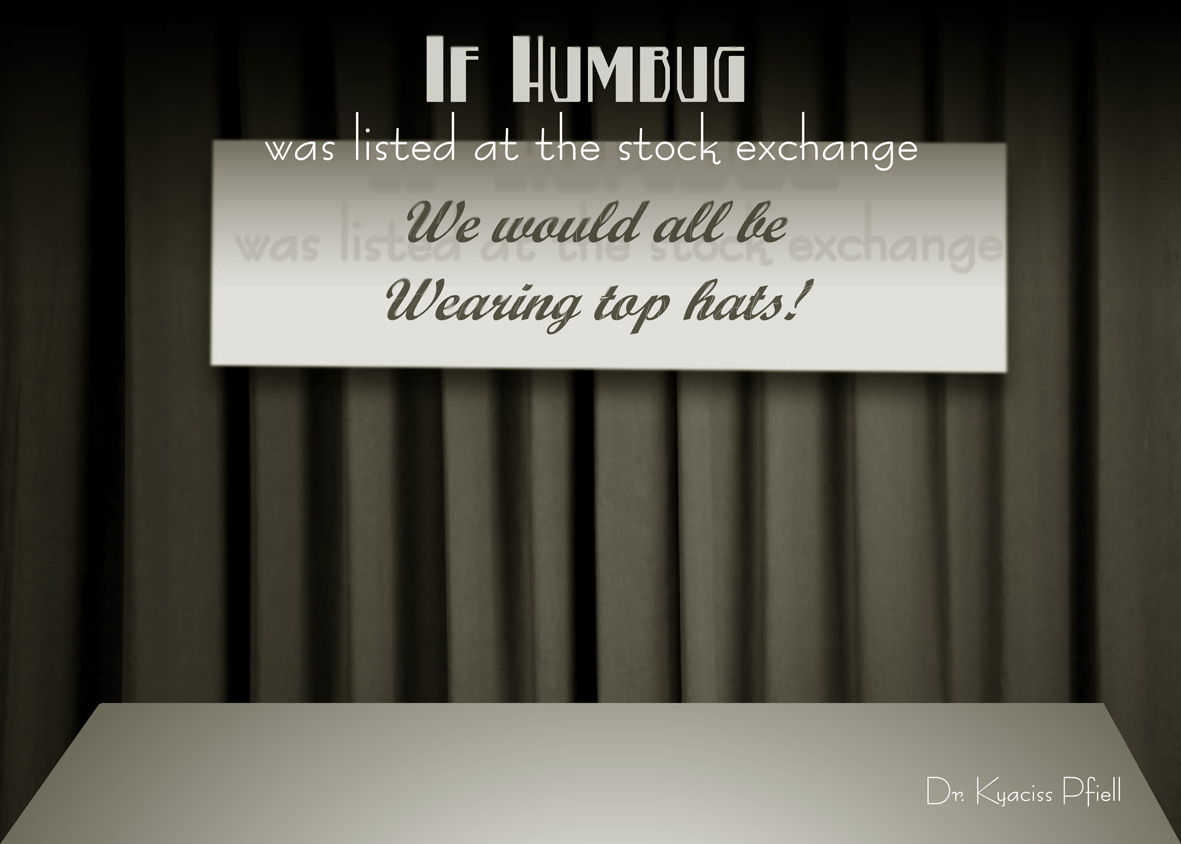The black and white digital image features a stage at the bottom, which appears slightly off-white, with a curtain in the background. The scene has a perspective effect, making the stage look narrower towards the top and wider towards the bottom. At the very top, in white text, it reads, "If Humbug was listed at the Stock Exchange." Below this text, in a white rectangular banner that stretches across the curtain, it says in black cursive, "We would all be wearing top hats!" This banner includes a drop shadow effect, giving depth to the text. In the bottom right corner, the name "Dr. K-Y-A-C-I-S-S P-F-I-E-L-L" is printed in fine white letters.